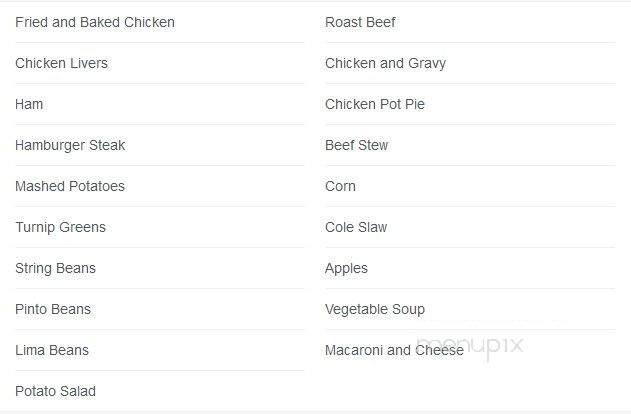The image displays a printed menu divided into two columns, each with its own tab, denoting various types of food. The top of the menu carries a faint watermark reading "menu PIX." The first column lists: fried and baked chicken, chicken livers, ham, hamburger steak, mashed potatoes, turnip greens, string beans, pinto beans, lima beans, and potato salad. The second column features: roast beef, chicken and gravy, chicken pot pie, beef stew, corn, coleslaw, apples, vegetable soup, and macaroni and cheese.